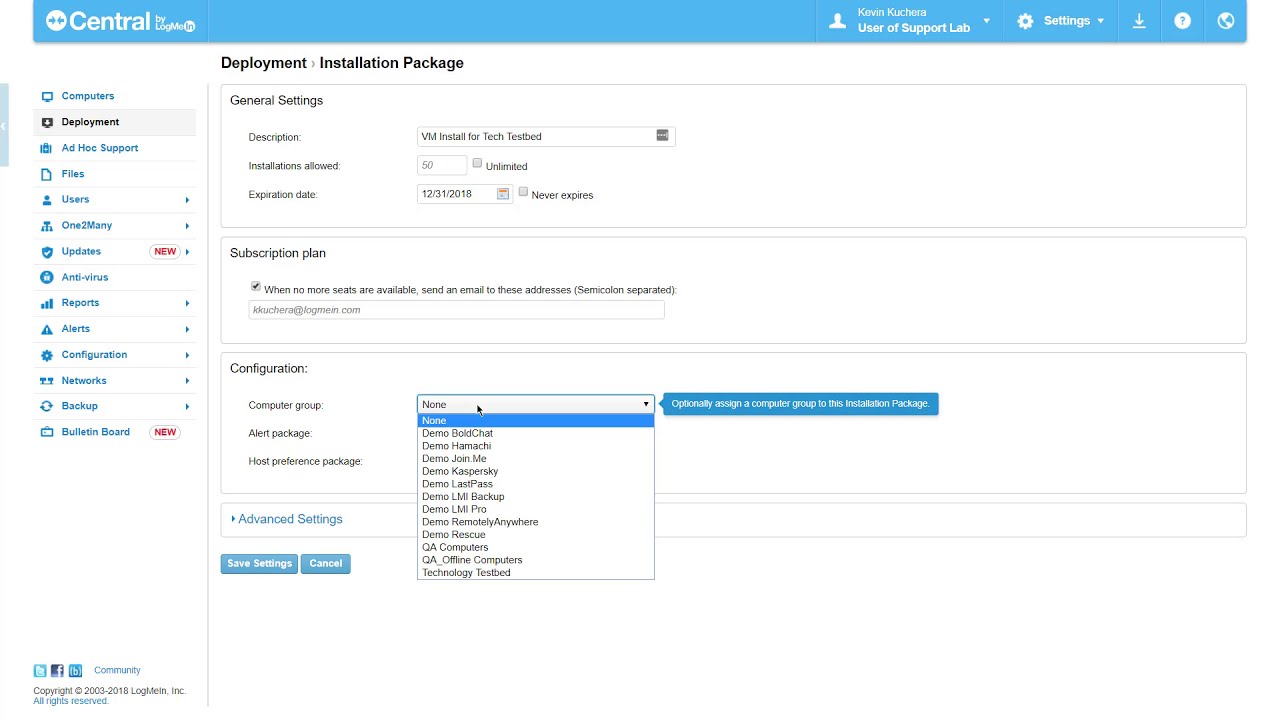In the image, a screenshot of a website or app interface is displayed against a white background. The top section features a baby blue banner stretching from left to right, with white fonts and icons. On the left side of the banner, there's a white circle with blue squiggly lines, followed by the word "central" in white text. Next to "central," the text "by LogMe" appears in smaller white font, and a white circle icon with "IN," suggesting a LinkedIn integration. 

Further right, there is a silhouette icon of a person's head and shoulders with the text "Kevin Kuchera" beneath it, all in white font. Below Kevin's name, the text "User of Support Lab" is displayed, accompanied by a dropdown arrow. Adjacent to this section, there's a cog wheel icon labeled "Settings" with a dropdown option, a download arrow icon with a horizontal line, and a white help icon featuring a question mark. Additionally, there's an earth silhouette icon.

Below the banner, a menu is present on the left side, with various clickable options in blue text, except for "Deployment" which is in black. The menu items, from top to bottom, are: Computers, Deployment, Ad Hoc Support, Files, Users, One to Many, Updates (with a "new" tag on the right), Antiviruses, Reports, Alerts, Configuration, Networks, Backup, and Bulletin Board (with another "new" tag). Each item is paired with corresponding icons.

To the right, the main content area starts with "Deployment" in black, followed by "Installation Package" and a thin line separating three boxes. Below "Deployment," lighter text reads "General Settings," and further down are sections labeled "Description," "Installation is Allowed," and "Expiration Date." In the "Description" box, it reads "VM installed for test tube or test bed." The "Installation is Allowed" field has "50," with an adjacent label "or unlimited." Under "Expiration Date," a box displays "12-31-2018" with a checkbox for "Never Expires."

A new section below includes a box labeled "Subscription Plan" at the top left with a checked checkbox. It instructs to send an email when no more seats are available, with a field for email addresses, showing "jkuchin at logmean.com."

The last box is "Work Configuration" in larger black font, containing "Computer Group," "Alert Package," "Host Preference Package." At the bottom, the text "Advanced Settings" appears in larger blue font, with two buttons "Save" and "Save and Settings" in white text against a baby blue background, next to a "Cancel" button. On the right, a large dropdown box shows "None" selected, with options including "Demo," featuring various computer programs like Kaspersky and LastPass.